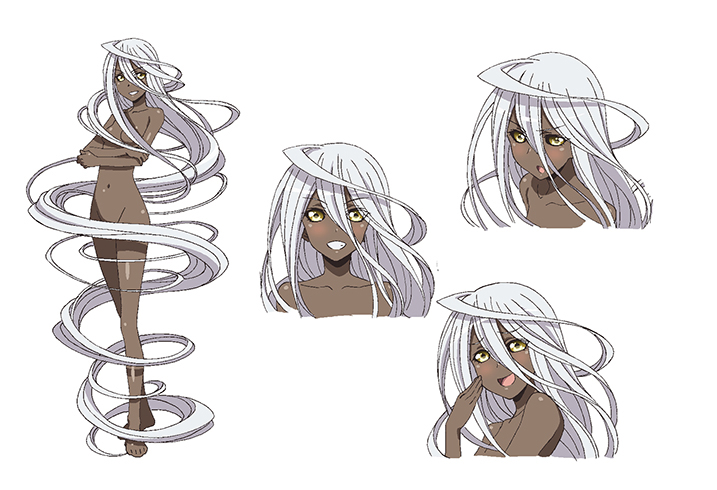This detailed image features an anime-style character depicted in four different drawings. On the left, she stands naked with deeply tanned, brown skin, but is modestly covered by her long, white hair that spirals around her body, reaching down to her toes. Her arms are crossed in front of her, and she gazes directly at the viewer with large eyes, likely brown with white reflections, and a confident demeanor.

To the right of this central figure are three additional images, each portraying the character from the shoulders up, with consistent white hair cascading around her face. The uppermost right image captures her with a shocked expression, mouth slightly agape as if she can't believe something she's seeing. The middle right image features a similar headshot where she has large eyes and an open-mouth smile, displaying her white teeth. The lowest image on the right shows her looking directly ahead and laughing, her hand raised near her cheek, with a visible pink tongue and an expression that exudes joy.